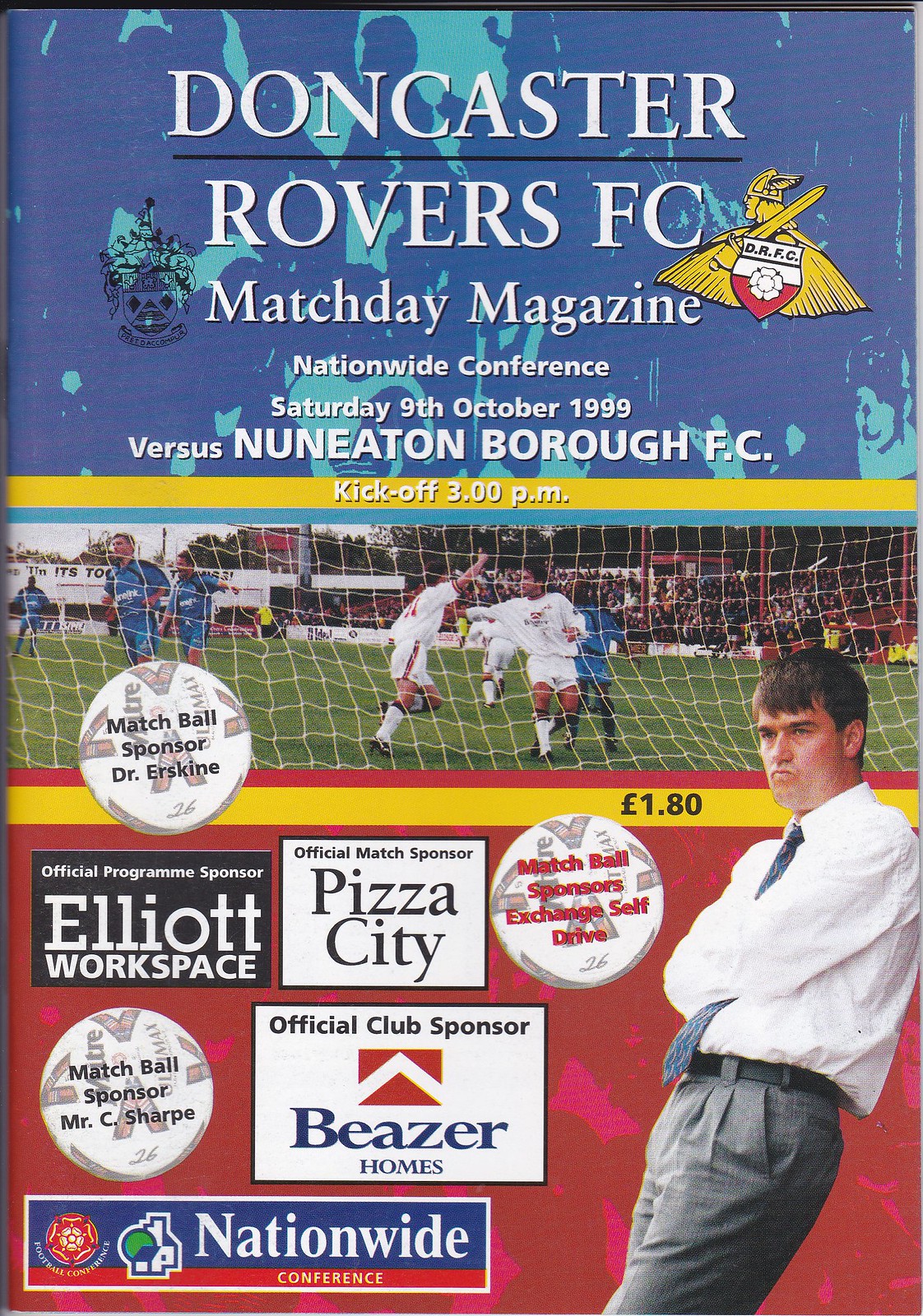The cover of the Matchday Magazine prominently features the logos of Doncaster and Rovers FC at the upper corners, with "Doncaster Rovers FC" in bold white lettering set against a light blue background. The central part of the image showcases an exciting in-game photo of soccer players celebrating on the pitch, viewed through a goal net, with a soccer ball in action. The ball displays the sentence "Matchball Sponsor Dr. Erskine." Additionally, two other circles highlight Match Ball Sponsors: Exchange Self-Drive and Mr. C Sharp. Detailed text informs readers of the Nationwide Conference match against Nuneaton Borough FC on Saturday, October 9th, 1999, with a 3 PM kickoff. The magazine is priced at £1.80. The lower part of the cover is filled with various advertisements, and to the right of these, a serious-looking man in a suit, arms crossed, is posed with a determined expression. The official club sponsors Beezer and Nationwide are also mentioned, completing the detailed and vibrant design.